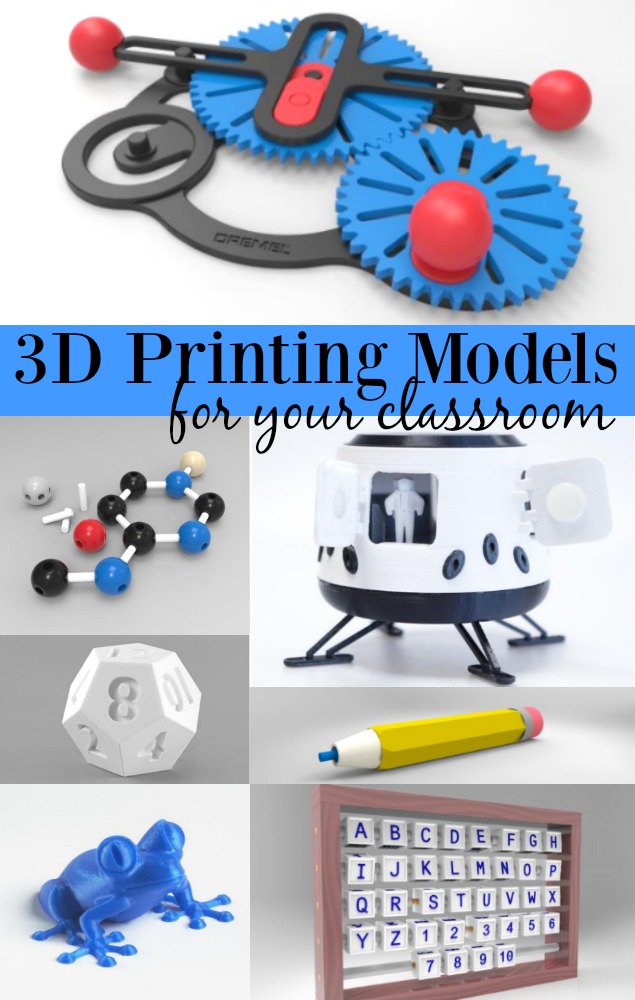**Detailed Caption:**

This portrait-oriented image collage consists of various smaller images arranged thoughtfully. At the very top, there is a white backdrop showcasing a black, red, and blue tool marked by intricate cogs and wheels. Beneath this is a striking blue bar adorned with bold, black text that reads "3D printing models for your classroom." 

Below the header, the image is divided into two columns, each containing three images. 

- **Top Left:** Set against a gray background, this image displays a molecular model composed of red, blue, black, white, and gray spheres interconnected by small, white rods.
- **Middle Left:** Showcases a multifaceted white die with numbers intricately carved into its surface.
- **Bottom Left:** Features a detailed, green 3D-printed frog.

- **Top Right:** Displays a monochrome black and white spaceship with an astronaut visible in the window.
- **Middle Right:** Highlights a vibrantly colored pencil embellished in yellow, white, blue, pink, and silver.
- **Bottom Right:** Contains a brown wooden frame holding alphabet letters in blue on white backgrounds, coupled with blue numerals one through ten.

This detailed and visually appealing layout effectively promotes diverse 3D printing models suitable for educational settings.